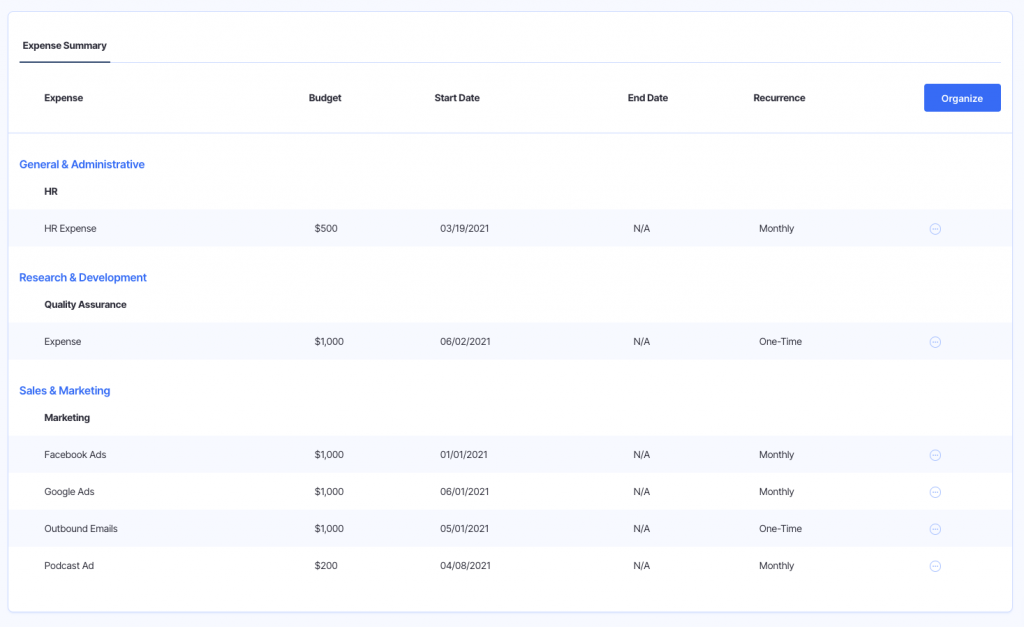This image is a screenshot of an expense summary screen, detailing various expenses and their associated budgets, timelines, and recurrence intervals. 

At the top left, the title "Expense Summary" is displayed in black font, followed by column headers: "Expense," "Budget," "Start Date," "End Date," and "Recurrence," respectively. A blue button with white text labeled "Organize" is positioned to the right of these headers.

The main section is divided into different categories, each highlighted in blue font. The first category, "General Administrative," lists an HR-related expense: "HR Expense" with a budget of $500, no specified end date, and a monthly recurrence.

Further down, "Research and Development" is followed by "Quality Assurance," under which an expense of $1,000 is listed, with no end date and a one-time recurrence.

The final section, "Sales and Marketing," includes various sub-expenses under "Marketing." These are: "Facebook Ads" with a $1,000 budget and a monthly recurrence; "Google Ads" with a $1,000 budget and a monthly recurrence; "Outbound Emails" with a $1,000 budget and a one-time recurrence; and "Podcast Ad" with a $200 budget and a monthly recurrence.